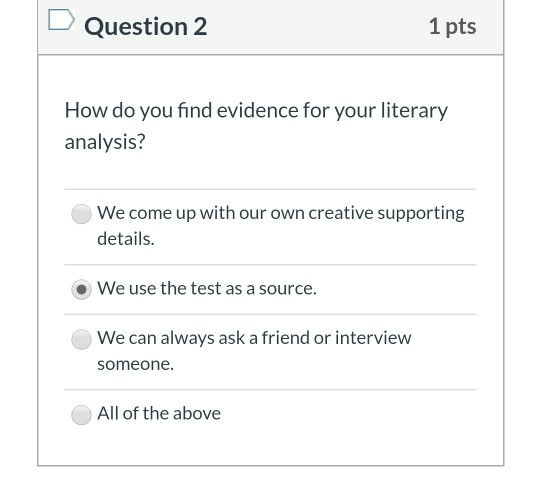The image depicts a quiz question presented within a square-shaped box. At the top of the square, a light gray banner features a smaller square that extends upward before tapering to a point. Within this banner, the text "Question 2" is prominently displayed, with the "Q" capitalized and the numeral "2" in dark print. To the right, it is indicated that the question is worth "1 pt," where "pt" is lowercase. 

Below the banner, the main question appears on a white background with black print that is slightly shaded in gray. The question reads: "How do you find evidence for your literary analysis?" and is followed by a question mark. Underneath the question, there is a horizontal line, followed by four answer choices. 

1. "We come up with our own creative supporting details."
2. "We use the test as a source."
3. "We can always ask a friend or interview someone."
4. "All of the above."

Each answer choice is prefaced by a small circle. The second answer choice, "We use the test as a source," is selected, indicated by a black dot filling the corresponding circle.